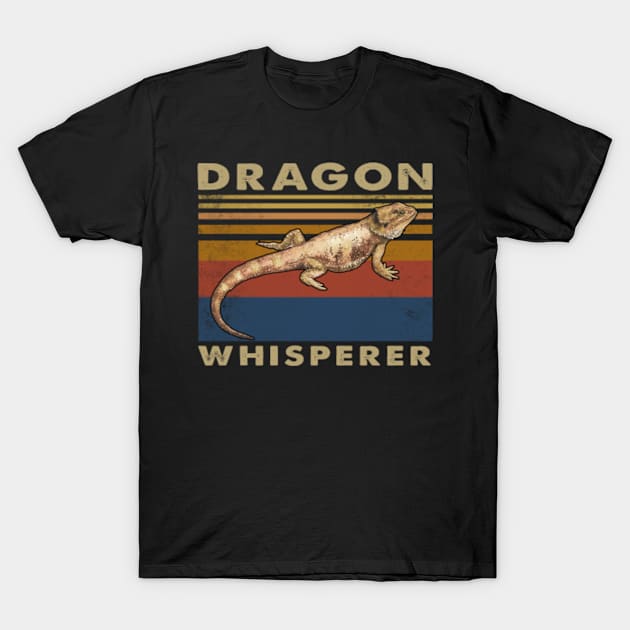This image features a black, short-sleeved, crewneck t-shirt with the words "Dragon Whisperer" screen printed on the front. The text "Dragon" appears at the top, and "Whisperer" is at the bottom. Centered on the chest is an illustration of a Komodo dragon, which is looking up toward the upper right. The lizard is primarily brownish-orange in color with stripes on its tail that curves down and to the left, then back to the right. Surrounding the Komodo dragon are multi-colored stripes that vary in width and color, including blue, orange, red, yellow, and green. The style of the image is that of a product photograph, showcasing the design and details of the t-shirt.